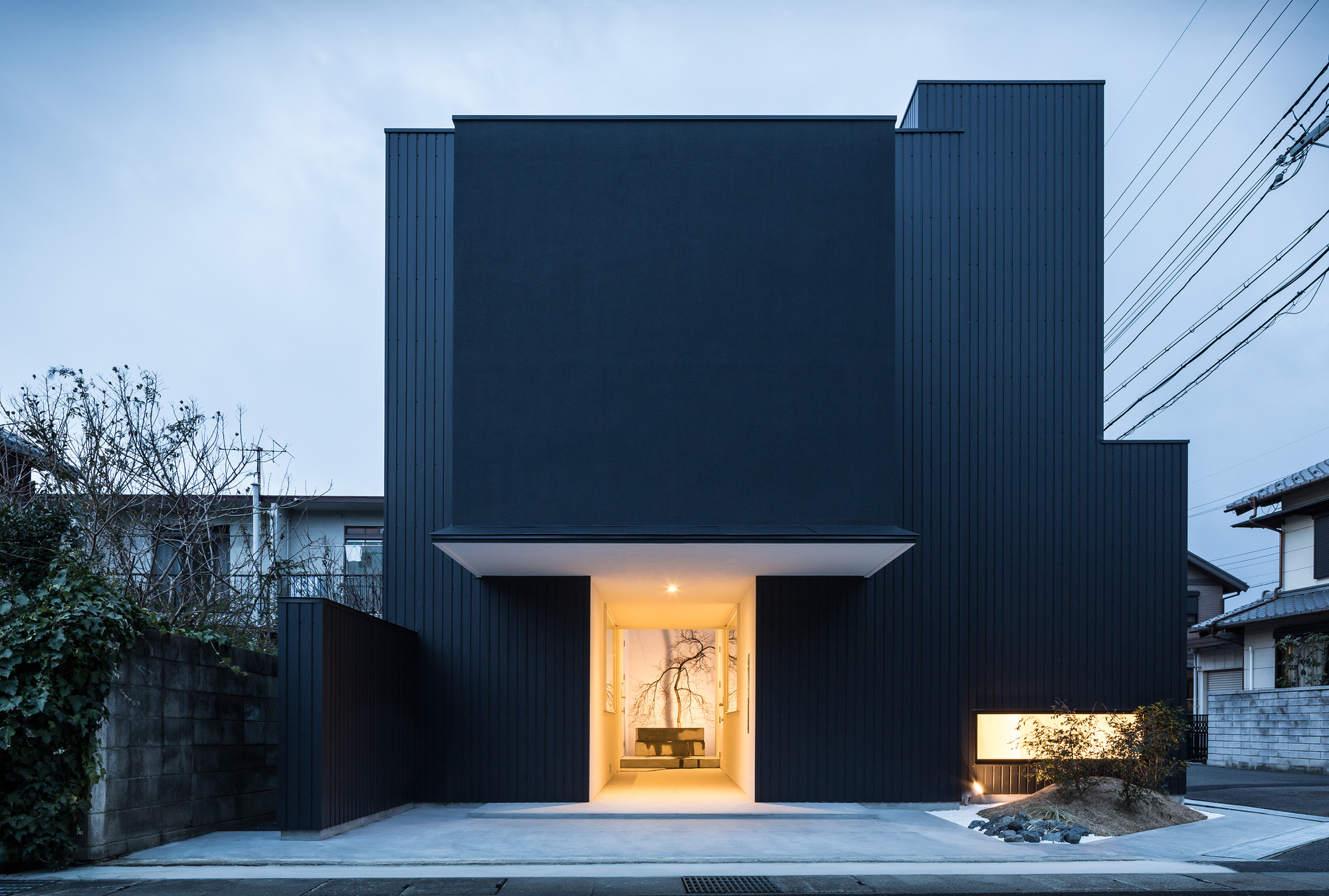The image depicts a striking, modern square building with a front portion painted in white at the bottom and a darker gray for most of its structure. It consists of a smaller cube with an overhang above the entrance and a larger cube behind. The front façade features black line paneling and a corridor with warm lighting that may display seating and tree branch artwork. A small wall made of concrete extends outward from the left side of the building, adorned with green vines and leafless shrubs suggesting seasonal changes. On the right, the structure has a taller rectangular section rising above the main building. 

In the foreground, a gray concrete lot and sidewalk are visible, bordered by a mound of soil with two small plants and stones. A road runs along the bottom and right side of the image, with traditional, old-looking buildings possessing weathered blue paint flanking the scene. The right side shows a secondary structure resembling a miniature brown house. 

Above, a network of power lines cuts across a gray sky, adding to the urban setting. On the left side, vegetation grows along a concrete wall, enhancing the juxtaposition between nature and modern architecture. There is no visible door, adding an abstract or monumental feel to the building, with a possible golden sign indicating it may function as a monument rather than a residential house.